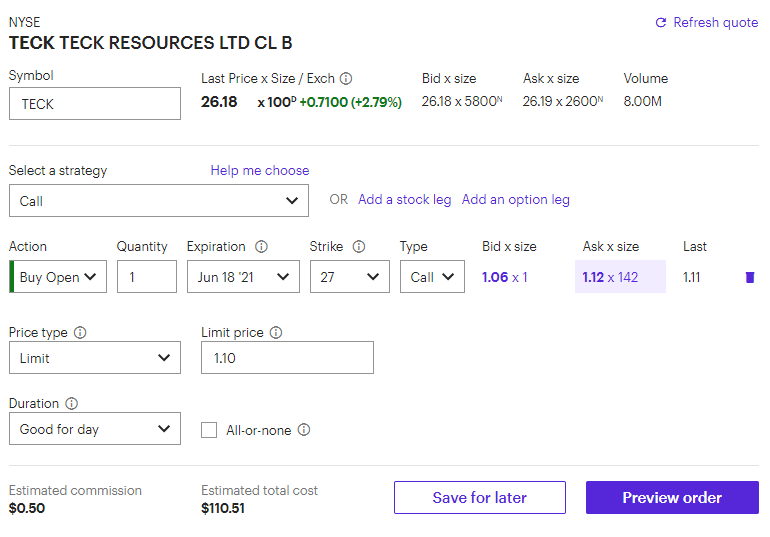This screenshot displays a pop-up menu with a white background, providing stock information. In the top left corner, the label "NYSE" is printed in gray font, and directly beneath it, "Tech Tech Resources LTD CLB" appears in bold black font. On the top right corner, there is a blue refresh icon accompanied by the text "Refresh Quote."

Beneath this section, a small white rectangular area with a faint black line displays the word "Symbol." Directly below this, a black-outlined rectangle contains the text "Tech." Adjacent to this, the information "Last Price X Size / EXCH" is listed, followed by stock details: "26.18 X 100 +0.7100 (+2.79%)," with the final part in green font indicating a price increase.

Further down, next to "Bid X Size," it reads "26.18 X 5800," while next to "Ask X Size," the text "26.19 X 26600" is shown.